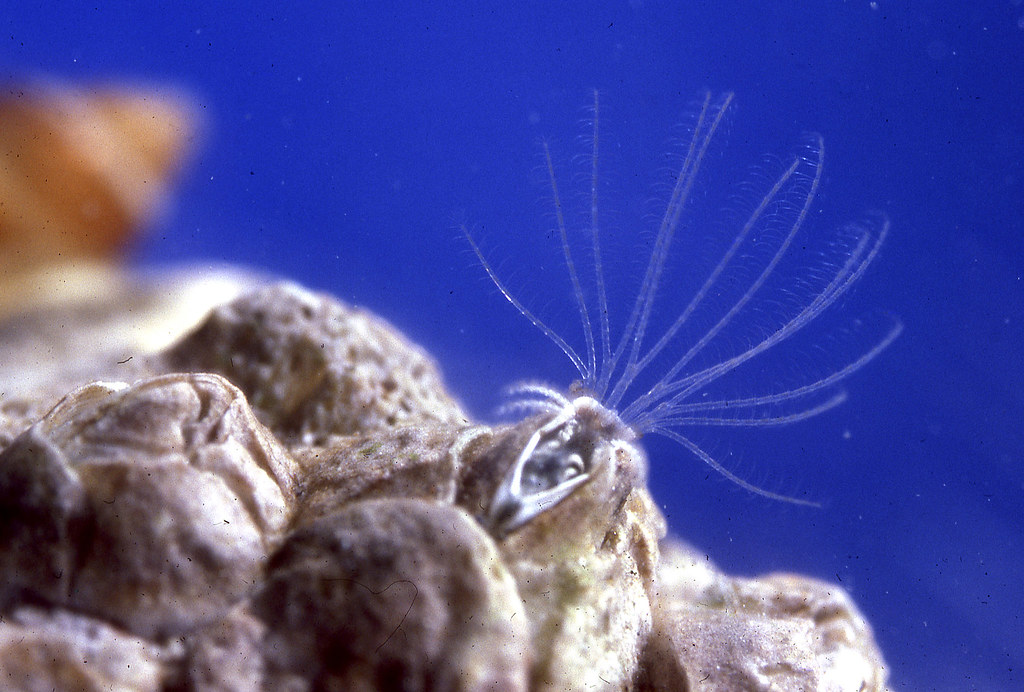This horizontally aligned, rectangular underwater image captures a vibrant scene with a blend of intriguing colors and forms. The upper part of the picture features various shades of blue, transitioning from a deeper blue on the left to a brighter blue on the right. On the upper left, there's a blurry, conical, and twisted orange shell with a white stripe looping around it. The central focus of the image is a wide, brownish object that appears to have numerous clear, grayish fibers or whiskers—roughly twelve in total—fanning out from it. Surrounding this central object, especially towards the bottom and left areas of the image, are large, bumpy, brownish-beige formations that resemble coral. Among these formations, there appears to be another piece of sea life, possibly embedded in the coral, which looks like an onion-shaped, whitish-gray organism with light brown accents. This intriguing sea creature looks to have elongated, transparent antennae with tiny hairs. Despite the grainy and blurry quality of the image, the dynamic underwater scene showcases the unique and vivid elements of marine life.